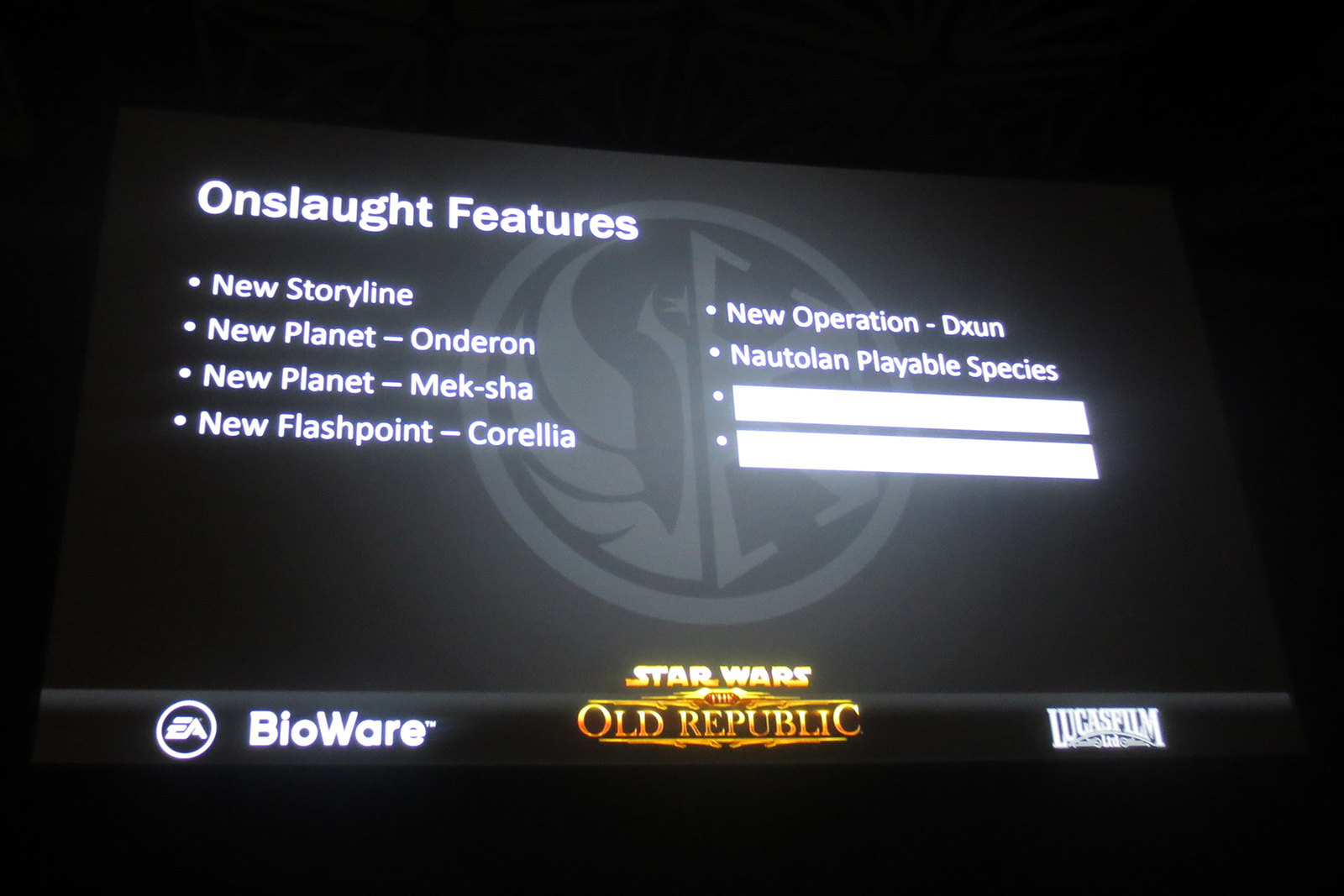The screenshot captures a computer monitor or television displaying the interface of the video game "Star Wars: The Old Republic," developed by BioWare and EA, with Lucasfilm Ltd. also credited. The screen's background features a dark gray hue with a lighter gray, round symbol containing elements resembling a half wing and an oddly shaped star split down the middle. Superimposed on this background is a menu titled "Onslaught Features." The menu lists various updates including a new storyline, new planets Onderon and Meksha, a new flashpoint on Corellia, a new operation on Dxun, and the introduction of the Natolian playable species. Additionally, in the bottom left corner, the logos for EA and BioWare are visible, while the center displays the game title "Star Wars: The Old Republic," and the bottom right corner features the Lucasfilm Ltd. logo.